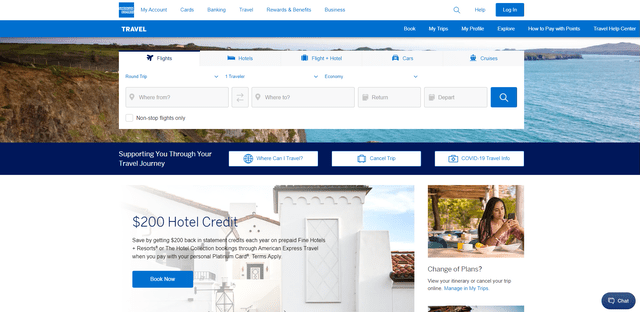The image appears to be a screenshot of a comprehensive online platform designed for flight information and travel-related services. In the upper left corner, there's a slightly blurry blue square containing white text, which is illegible. Adjacent to this are clickable blue text links labeled "My Account," "Cards," "Banking," "Travel," "Rewards & Benefits," and "Business." Towards the right side, there is a blue square for logging in.

Prominently displayed in white text is the word "Travel," situated above a wide, slender rectangular image that spans the entire width of the page. This scenic image depicts a dramatic landscape featuring a cliff adorned with lush greenery on the left and right, seamlessly transitioning into expansive ocean waters dotted with distant islands.

Above this captivating image, there is a functional white search box titled "Flights." This box includes fields for inputting travel details: "Where From," "Where To," "Return," and "Depart," accompanied by a blue magnifying glass icon on the right for initiating the search.

Beneath the search box, an advertisement offers a $200 hotel credit, promoting the benefit of receiving $200 back in statement credits each year on prepaid bookings at fine hotels and resorts. A clickable "Book Now" button accompanies this offer.

In the lower right corner of the webpage, there is an image of a woman dining at a table, seemingly enjoying a vacation with trees visible in the background. Adjacent to her image, text invites users to manage their travel plans with the options to "View Your Itinerary" or "Cancel Your Trip Online," followed by a clickable "Manage My Trips" button in blue.